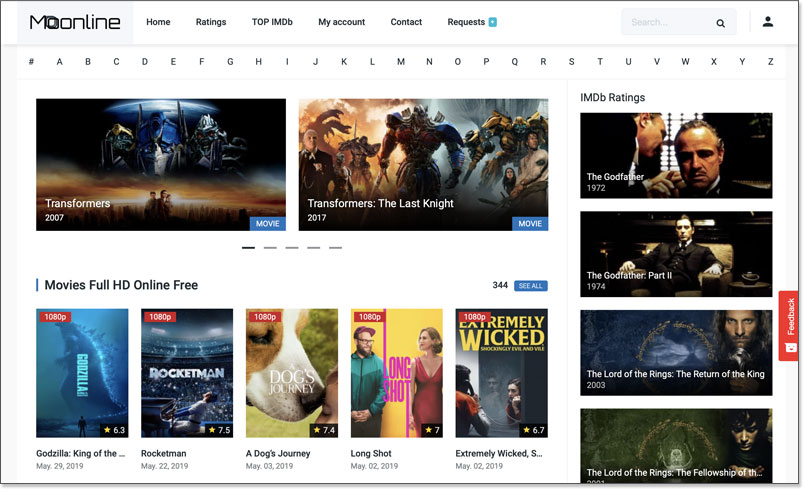In this screenshot of a website, the upper left corner features a gray box with the text "Moonline". Adjacent to this, the rest of the header is white with a navigation menu that includes the following buttons, from left to right: "In Buttons", "Home", "Ratings", "Top IMDB", "My Account", "Contact", and "Requests". At the upper right corner, there's a gray search bar with a black magnifying glass icon.

Below the header, there is a white banner displaying the letters A through Z. Beneath this, a selection of movie thumbnails is visible. The top left thumbnail shows "Transformers 2007", with "Transformers: The Last Knight" positioned to its right. Just below these thumbnails, a bold header reads "Movies Full HD Online Free". The movies featured in this section, from left to right, include "Godzilla", "Rocketman", "A Dog's Journey" (with an image showing a dog's snout touching a child's face from the upper left corner), "Long Shot", and "Extremely Wicked".